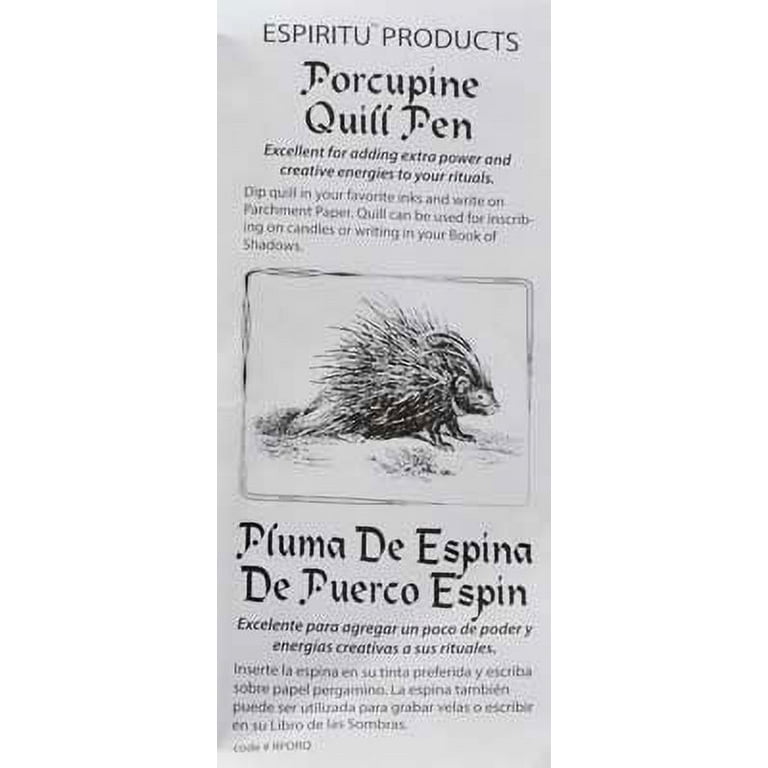The image is a black and white flyer for a porcupine quill pen by Espiritu products. Centrally, there is a detailed hand-drawn illustration of a porcupine encased in a simple square border. Above the drawing, black text reads, "Espiritu Products Porcupine Quill Pen," followed by a description: "Excellent for adding extra power and creative energies to your rituals. Dip quill in your favorite inks and write on parchment paper. Quill can be used for inscribing on candles or writing in your book of shadows." Below the drawing, there is the same information provided in Spanish, beginning with "Pluma de Espina de Puerco Espín." The text and image are set against a gray background, emphasizing the mystical and utilitarian uses of the quill pen for ritualistic purposes.